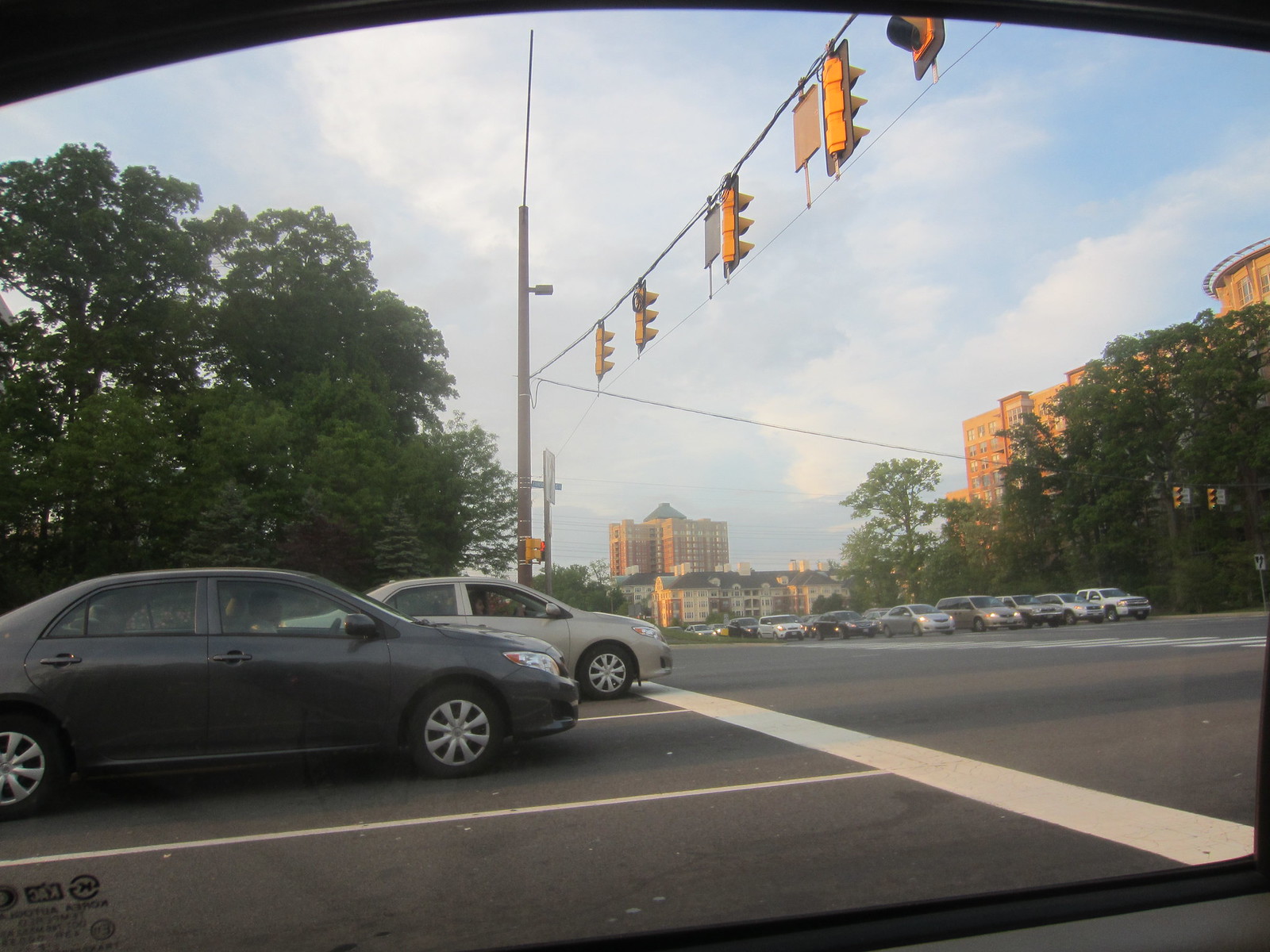This photograph captures the view from inside a vehicle, with the top edge of the image framed by the curved, black interior of the car window. A small portion of the car's interior is visible along the bottom of the image, including an unreadable section of text usually found on vehicle windows. The scene outside reveals a large, busy intersection. A traffic light pole and its attached wires stretch across the frame, supporting five yellow traffic lights, although their current signals are not visible. Adjacent to the photographer's vehicle is an empty lane, followed by two occupied lanes with dark gray and light gray sedans, respectively. Further into the intersection, five columns of cars, each extending about five rows back, wait for the traffic light to change. The backdrop includes buildings from a distant city skyline, bordered by large trees and bushes situated at each corner of the intersection. The sky overhead is dotted with wispy, fluffy clouds, allowing patches of blue sky to peek through, indicating a clear, daytime setting.